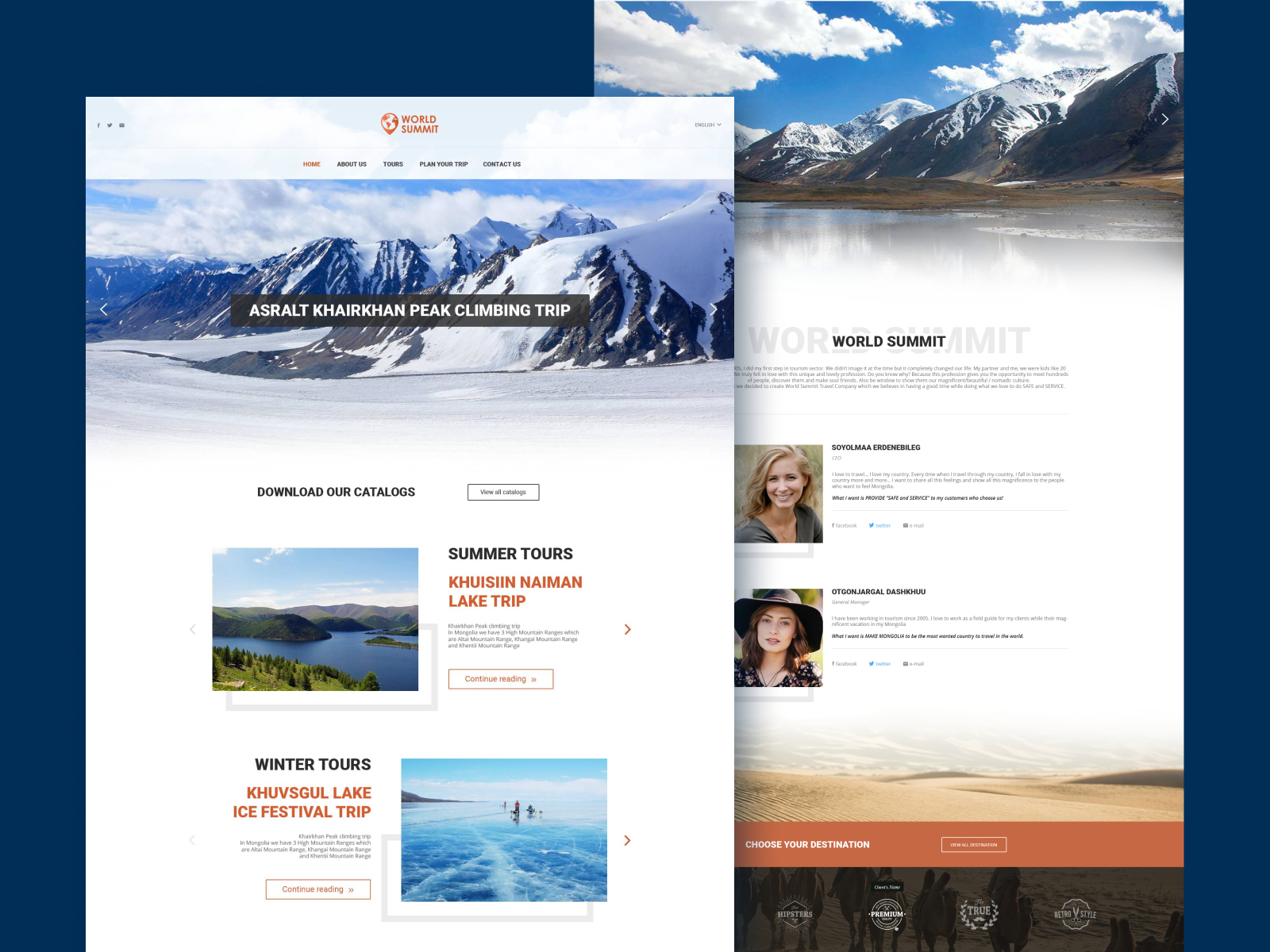The image appears to be an advertisement for an outdoor adventure event, likely featured on a website. The top of the advertisement showcases a striking photograph of snow-covered, rocky mountains set in a desolate area, devoid of trees or buildings, emphasizing the rugged and untouched nature of the landscape. Superimposed on this image is a black text box with white lettering that reads "ASRALT, Tarracan Peak Climbing Trip." 

Beneath this dramatic image is a section with a white background featuring a call-to-action in black text: "Download our catalog." Below, there are two additional images depicting different tour options. The first image portrays a serene summer scene and is labeled "Summer Tours," while the second image returns to a wintry landscape, labeled "Winter Tours." Each tour option includes a brief location description and a clickable box inviting viewers to "Continue reading about the trip," providing a clear pathway for users to explore further details. 

Overall, the advertisement uses vivid, contrasting imagery and clear, inviting text to draw attention to the various seasonal adventures offered.